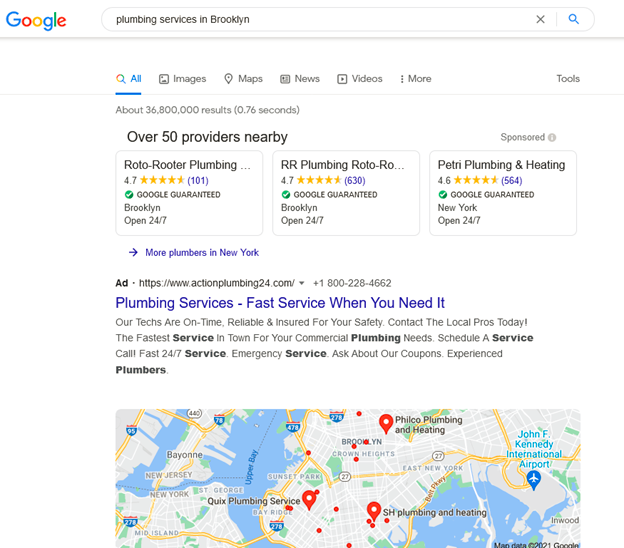Screenshot Description:

The screenshot features a Google search results page with a clean white background. In the upper left-hand corner, the Google logo is displayed in its signature colors. Adjacent to the logo on the right is a long oval search bar containing the query "plumbing services in Brooklyn" in black text. On the right side inside the search bar, there is a black “X” and a blue magnifying glass icon.

Directly below the search bar, a menu is presented with six options. The first option, "All," is highlighted in blue and underlined, while the following options—"Images," "Maps," "News," "Videos," and an ellipsis for more—are displayed in gray. To the far right of the menu, there is a "Tools" button.

Further down, the page indicates that there are about 36,800,000 results for the search query. A few lines below this, an indented line in bold black text states "Over 50 providers nearby."

The results section shows three horizontally aligned square boxes detailing service providers:
1. **Roto-Rooter Plumbing** with bold black text.
2. **RR Plumbing Roto-RO** with bold black text.
3. **Petri Plumbing & Heating** with bold black text.

Each of these listings includes a star rating and a "Google Guaranteed" badge, indicated by a green circle with white text on the left of each provider’s name. Their locations are specified as Brooklyn and Brooklyn, New York.

Below the provider listings, a blue right-pointing arrow and the blue text "More plumbers in New York" invite users to explore additional options. Following this, there is an ad section with the headline "Plumbing Services - Fast Service When You Need It," displayed in blue. This section provides further information about the service and is accompanied by a rectangular Google map at the bottom of the screenshot.